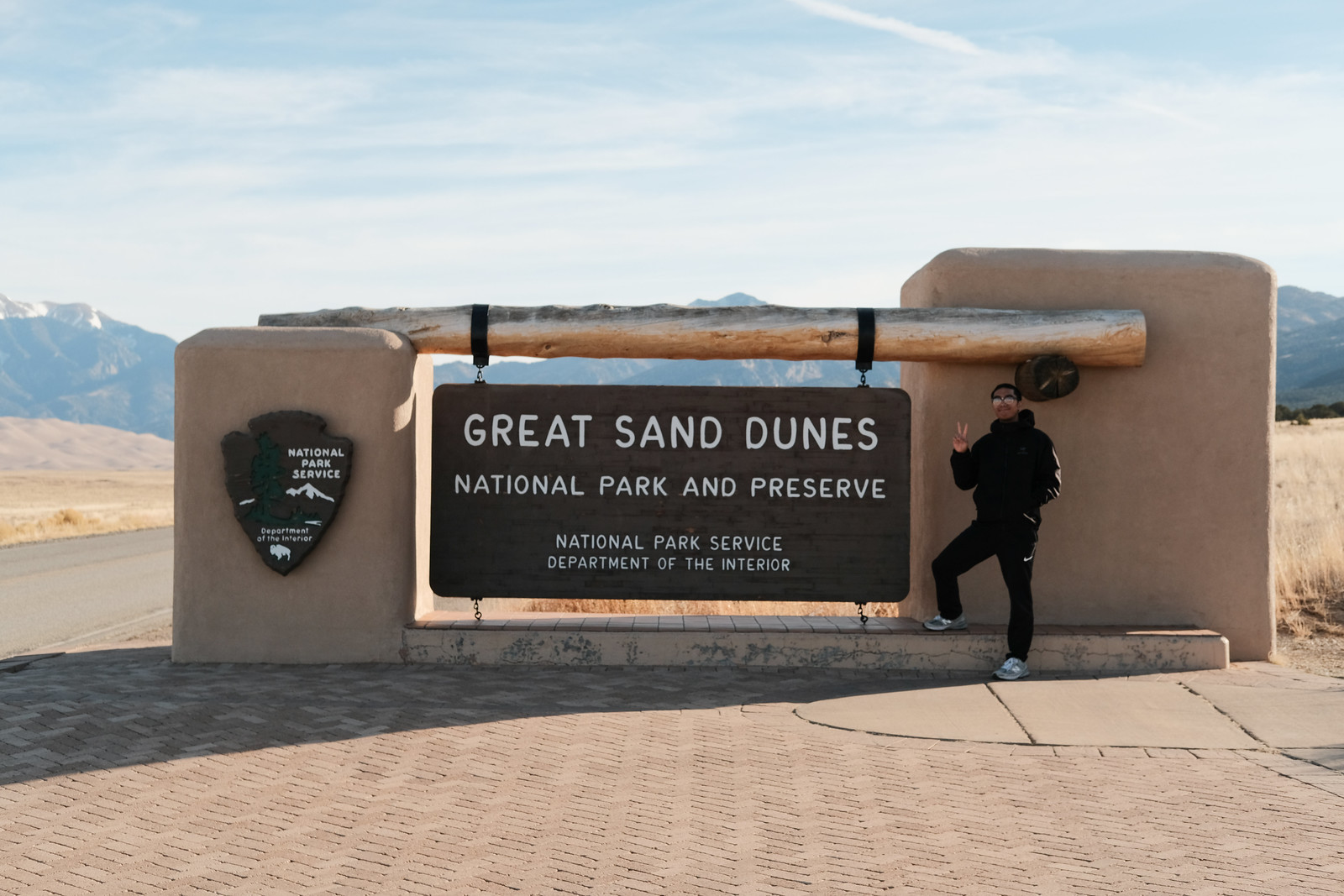This horizontally aligned rectangular outdoor image captures a scenic and informative view of the Great Sand Dunes National Park and Preserve entrance. At the top of the picture, the sky is a vivid blue adorned with numerous feathery white clouds. Dominating the middle portion is a large stone structure that serves as the backdrop for the park's signage. On the left side of the structure, a rectangular stone stands vertically with a National Park Service plaque, featuring an arrowhead design and a white buffalo emblem at the bottom. In the center, a prominent wooden log supports a sign that reads "Great Sand Dunes National Park and Preserve" in bold, white uppercase letters, along with "National Park Service, Department of the Interior" underneath.

On the right side of the image, a sizable stone pedestal stands, plain but sturdy, and a young man poses in front of it. He has short black hair and is dressed entirely in black, sporting a jacket, Nike pants, and white tennis shoes. He wears sunglasses and flashes a peace sign towards the camera. Below the stone structure, the foreground showcases a red or pink brick walkway, leading towards the left where a road is visible. In the background, the left side reveals majestic mountains with snow-capped peaks, adding natural beauty to the scene. Sporadic patches of grass are also noticeable, depicting the pristine environment surrounding the entrance.